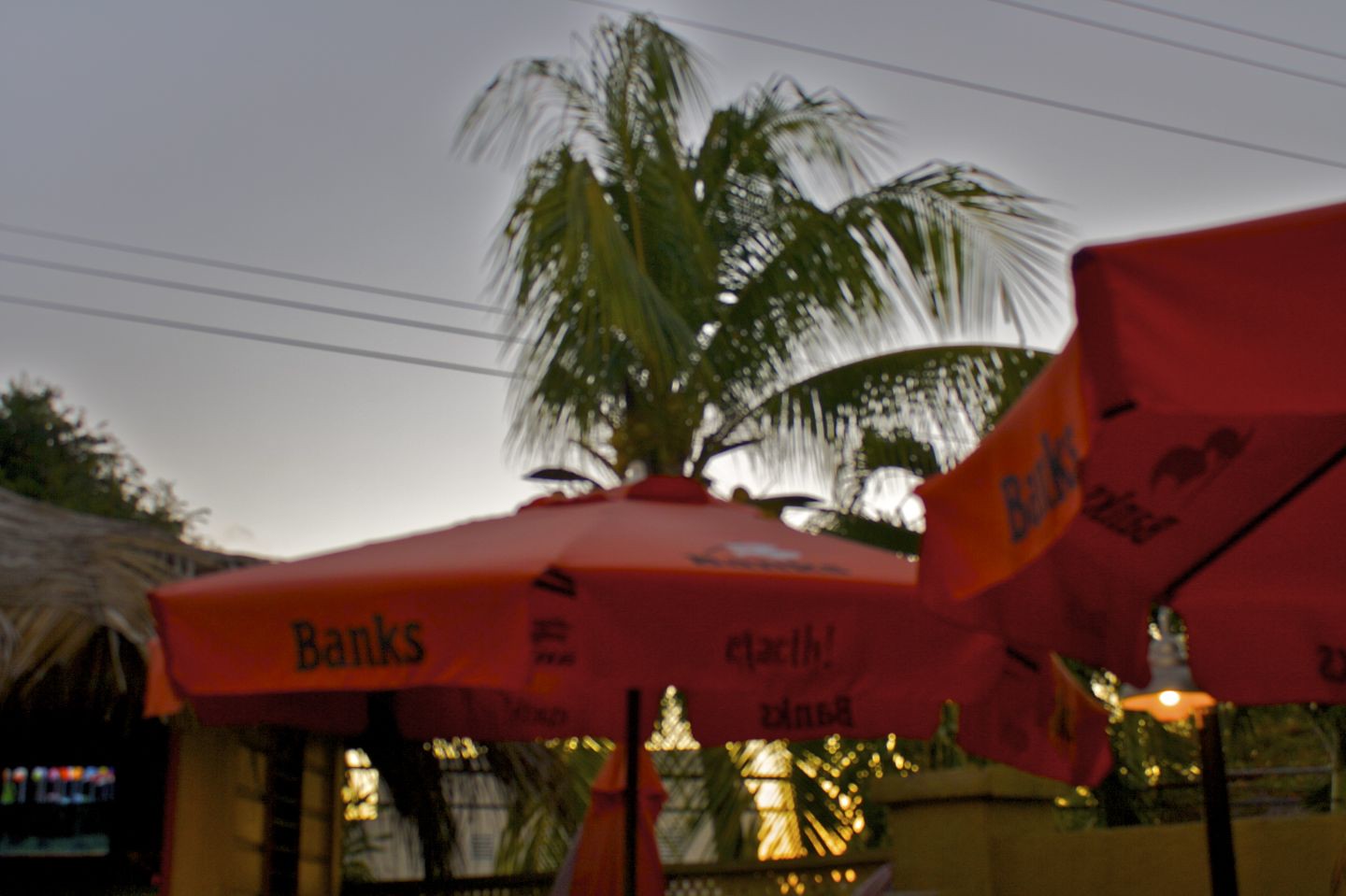The image captures a blurry, dusk scene at an outdoor café or restaurant in a warm climate, evidenced by the palm tree with leaves angled towards the bottom right. Two prominent red patio umbrellas in the center, printed with the word "Banks" in black text, dominate the foreground. A third umbrella behind them remains closed. The sky is a dark, stormy gray, creating an ominous atmosphere, suggesting impending rain. On the left, there's a hut-like building with a straw roof, housing a drink machine. The middle ground is illuminated by lights that cast a glow on a back fence. Overhead, telephone wires crisscross the sky, adding to the scene's layered details. The setting suggests a vibrant, albeit slightly chaotic, summer evening at a soon-to-be busy open-air dining spot.